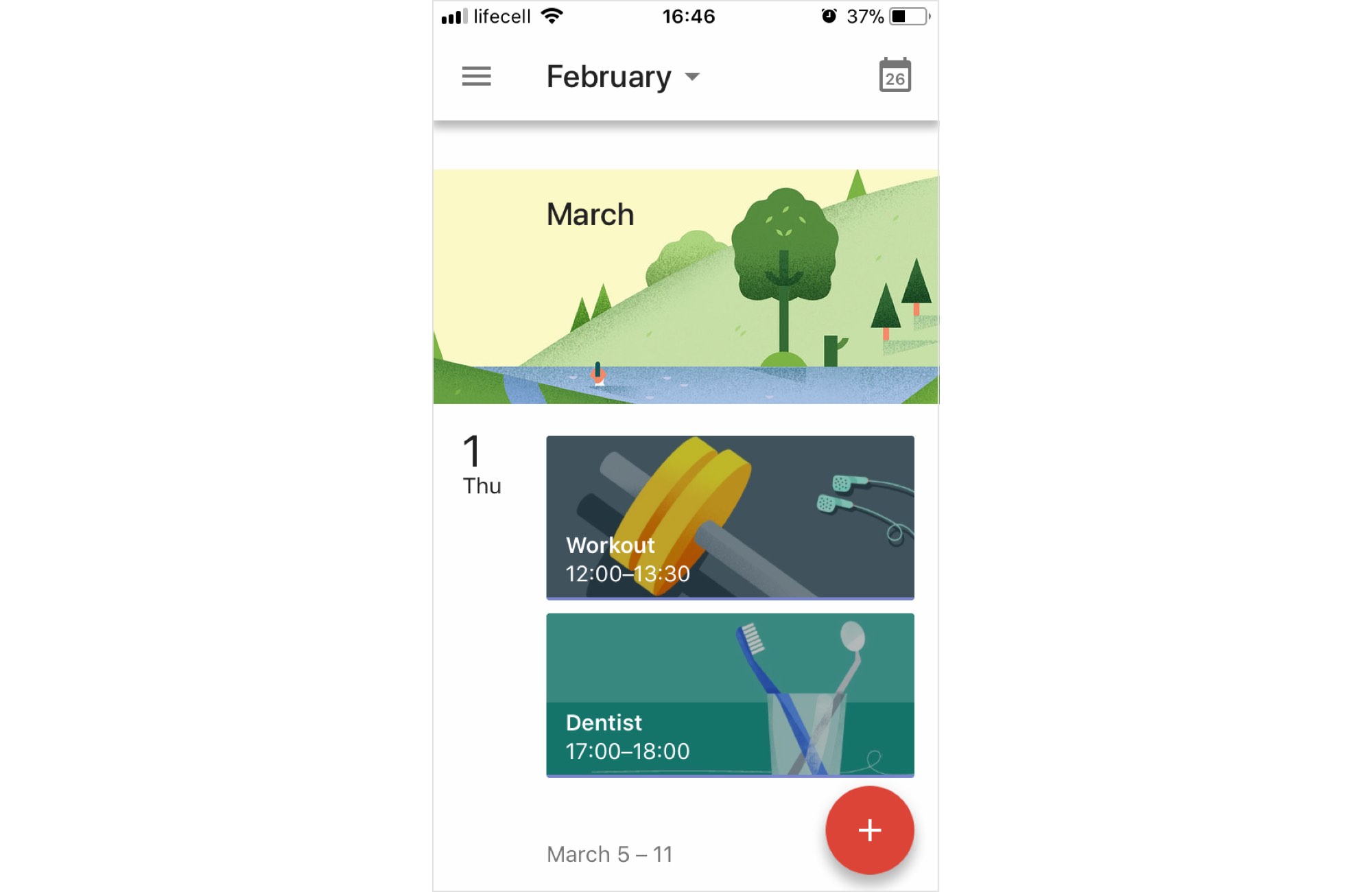The image is a partial screenshot of a planning or agenda-style application displayed on a mobile phone. In the upper right corner of the screen, the signal strength is shown with three of the four bars filled. To its right, the carrier name "lifecell" is written in lowercase letters, followed by a fully darkened Wi-Fi indicator. The time "16:46" is centered at the top of the screen, and to the left of the time is an alarm clock icon. Next to the icon, "37%" is displayed alongside a battery icon indicating the battery is not fully charged.

Below the status indicators, on the left side, there are three horizontal menu bars. Adjacent to this, the word "February" appears with a dropdown arrow next to it. On the far right, there is a stylized page-a-day calendar icon showing the number "26."

Further down, a graphic section titled "March" features a simplistic and angular drawing on a yellow background. The illustration depicts a hill with big green trees, stylized as simple triangles with trunks, and water in front of the hill. There is also an angular representation of a person in the water.

Below this graphic, the text "1" is displayed on the left, followed by "THU." To the right, a panel features a simple line drawing with shadow details of a barbell with two orange weights on a grey pole, next to stylized turquoise wired earbud headphones. This panel has a dark grey background with the text "Workout, 12:00 - 13:30" on top of it.

Below the workout section, a teal rectangular box displays a graphic image of a clear cup containing a blue toothbrush and a dentist's mirror. The accompanying text reads "Dentist, 17:00 - 18:00." At the bottom of the screen, "March 5 - 11" is shown, with a round red icon containing a white plus sign superimposed on top in shadow style presentation.